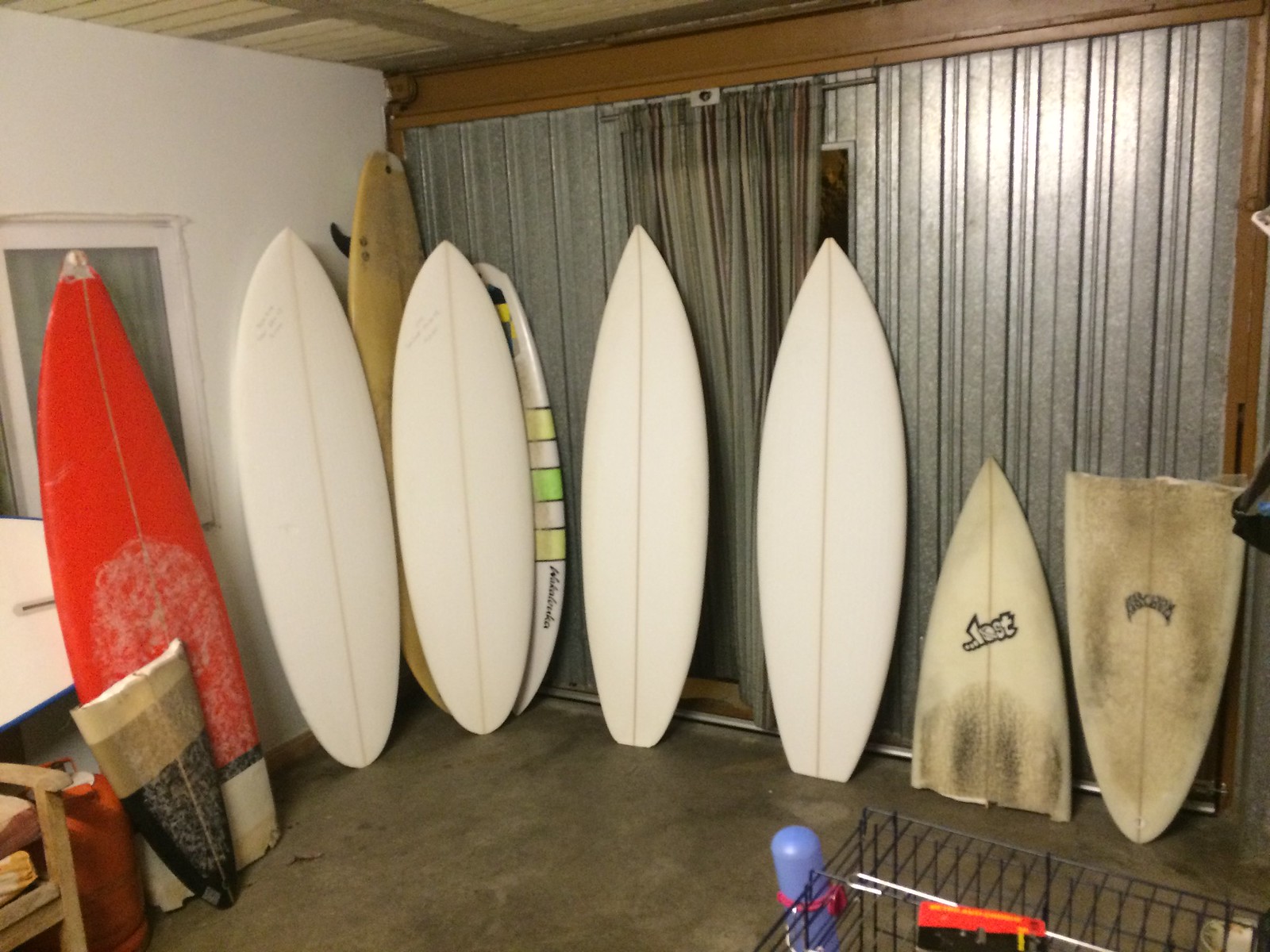Inside a room, possibly a garage or basement with a concrete floor, there are seven surfboards standing against the back wall. The majority of these surfboards are white, but there are also notable exceptions: a red surfboard on the far left and a white, yellow, and green-striped surfboard on the right. Among the collection, a broken surfboard lies in two pieces, heavily dirtied and split in half, sitting on the far right. Behind the surfboards, a long wooden board is present as well. There is a silver structure, possibly part of a garage door, visible behind some of the surfboards. Additionally, the room contains a small red bag, a white shelving unit to the left, a chair, and a cage on the lower right, potentially for a small animal. A curtain in the room seems to separate this space from the rest of the house.